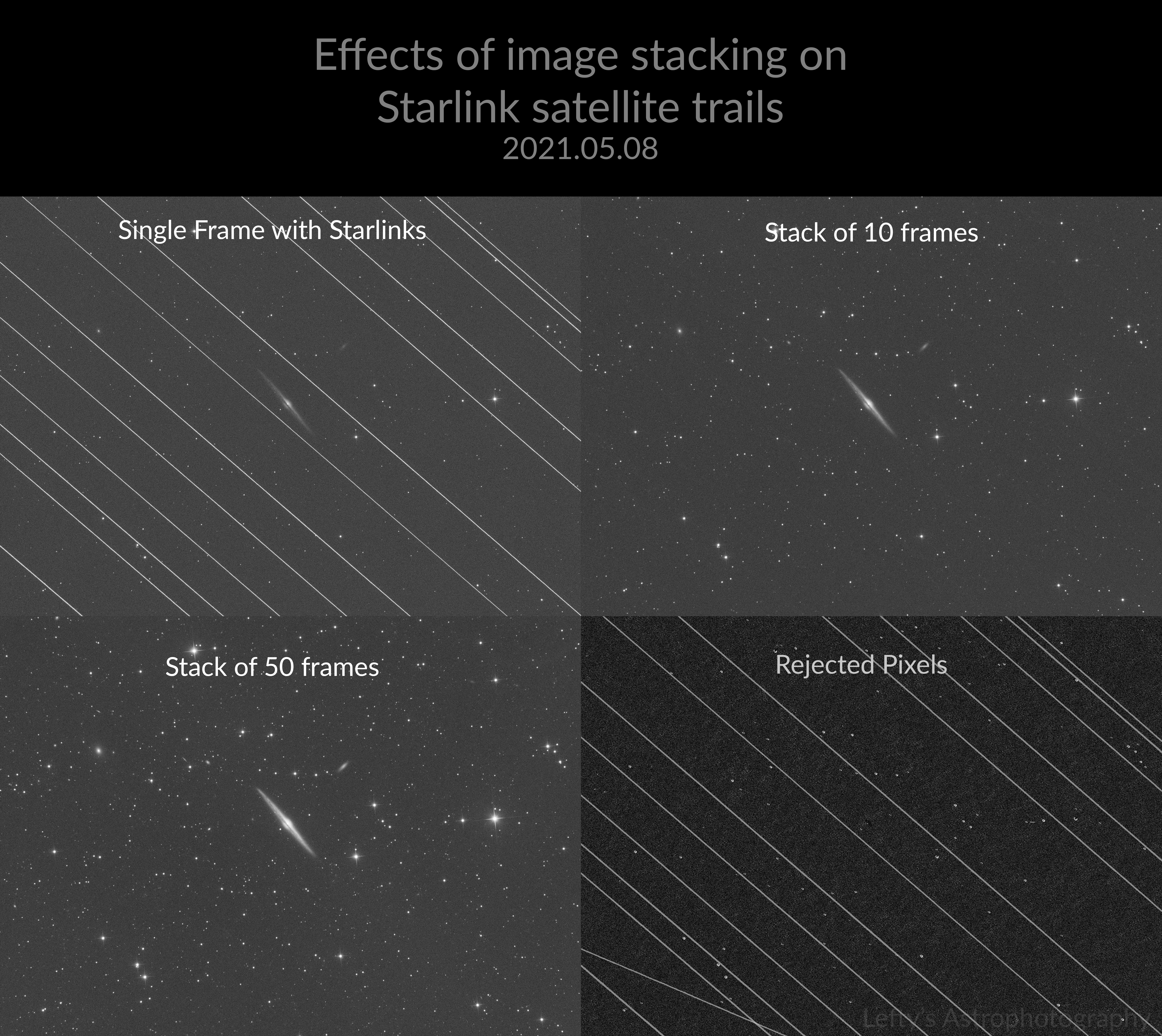Here is a detailed and cleaned-up caption for the series of images described:

---

**Title: "Effects of Image Stacking on Starlink Satellite Trails - 2021.05.08"**

This collage consists of four black and white photographs, each illustrating different effects of image stacking on visibility of Starlink satellite trails in astronomical images. 

**Top Header:** 
- The title is prominently displayed on a black background with white text: "Effects of Image Stacking on Starlink Satellite Trails 2021.05.08."

**First Panel (Top Left):**
- Caption: "Single Frame with Starlinks"
- Description: This image captures a single frame of the night sky. Diagonal trails from Starlink satellites streak across from the top left to the bottom right, creating numerous bright lines over the black and white expanse of space.

**Second Panel (Top Right):**
- Caption: "Stack of 10 Frames"
- Description: This photograph is a composite of ten stacked frames, showing the night sky without the intrusive satellite trails. The image features a clear, star-studded background, and includes visible stars and galaxies, highlighting the reduction in satellite interference.

**Third Panel (Bottom Right):**
- Caption: "Rejected Pixels"
- Description: This panel displays the pixels rejected during the stacking process. It features diagonal white lines against a darker space background compared to the other images. The stars, planets, and galaxies appear dimmer and more subdued, emphasizing the removed areas where satellite trails were present.

**Fourth Panel (Bottom Left):**
- Caption: "Stack of 50 Frames"
- Description: The final image is a detailed composite of fifty stacked frames. It does not show any diagonal satellite trails and offers an enhanced, zoomed-in view of the night sky. Stars appear more illuminated, and a spiral galaxy is prominently visible in the center, surrounded by smaller dots that represent other stars, planets, and galaxies.

---

This comprehensive caption provides clear and detailed information about each panel, aiding viewers in understanding the effects of image stacking on astronomical photography.